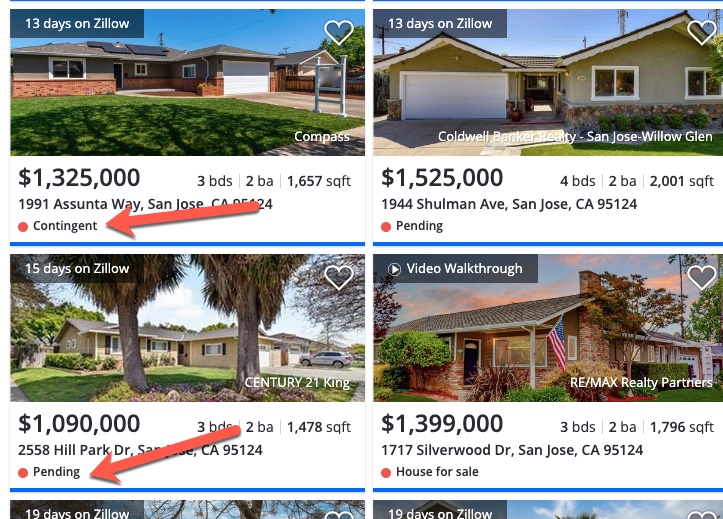This webpage displays various houses for sale, each with detailed descriptions and visual elements.

**Left Panel:**
- **House 1:**
  - **Appearance:** Brick with tan siding, white windows, and a gray roof featuring black solar panels.
  - **Listing Info:** Marked as "Contingent" within a red circle and a red arrow pointing to it. Priced at $1,325,000.
  - **Details:** 3 bedrooms, 2 baths, 1,657 square feet.
  - **Address:** 1991 ASSUNTA Way, San Jose, CA (ZIP partially visible, starts with 24).
  - **Realtor:** Compass (indicated in bold white text).

**Right Panel:**
- **House 2:**
  - **Appearance:** Olive green textured siding with white trim and garage, dark green peculiar grass and bushes.
  - **Listing Info:** Listed for $1,525,000 and marked as "Pending." Indicated as "13 days on Zillow."
  - **Details:** 4 bedrooms, 2 baths, 2,001 square feet.
  - **Address:** 1944 SHULMAN Avenue, San Jose, CA 95124.
  - **Realtor:** Coldwell Banker Realty, San Jose, Willow Glen.

**Lower Left:**
- **House 3:**
  - **Appearance:** Cream-colored siding with white trim and garage, black shutters, large weeping willow trees, a silver car in the concrete driveway, and dark green grass with hedges.
  - **Listing Info:** Listed for $1,090,000 and marked as "Pending." Indicated as "15 days on Zillow."
  - **Details:** 3 bedrooms, 2 baths, 1,478 square feet.
  - **Address:** 2558 Hill Park Drive, San Jose, CA 95124 (ZIP partially visible).

**Lower Right:**
- **House 4:**
  - **Appearance:** Brown and red brick house with a gray roof, white siding and supports, black door, and white garage. The sky is pink and blue with colorful green bushes.
  - **Listing Info:** Listed for $1,399,000 and marked with "House for Sale." Includes a "Video Walkthrough" feature, indicated by a white-bordered circle with a white triangle within a black rectangle.
  - **Details:** 3 bedrooms, 2 baths, 1,796 square feet.
  - **Address:** 1717 Silverwood Drive, San Jose, CA 95124.

This comprehensive display offers a range of homes with distinct features, pricing, and statuses, catering to potential buyers in San Jose, California.